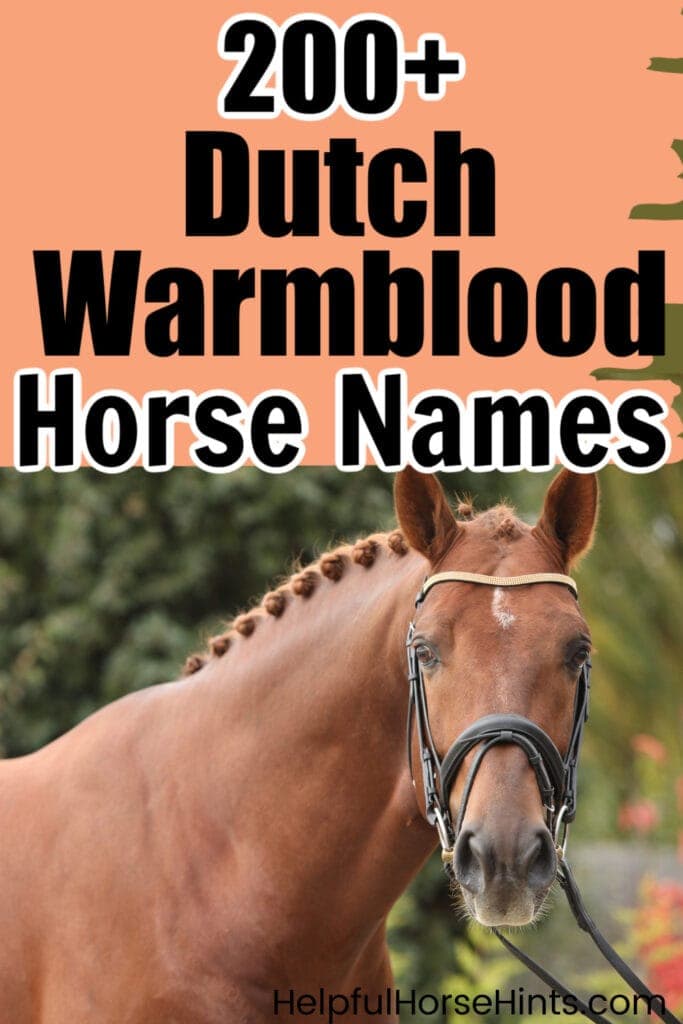The poster is a vertical rectangular design featuring a brown horse with braided hair, facing directly at the camera. The horse, adorned with a black leather bridle and a yellow strap on its forehead, is positioned towards the left side of the image. Its nose and mouth are also strapped by the black bridle. The background behind the horse is a blurry mix of green plants resembling trees, with red or pink flowers visible at the bottom right. The top half of the poster has a peach-colored background with text. It prominently displays "200 plus Dutch Warmblood Horse Names," with "200 plus" and "Horse Names" in black text, outlined in white, while "Dutch Warmblood" is in solid black. At the bottom right corner of the poster, the website helpfulhorsehints.com is noted in black text.